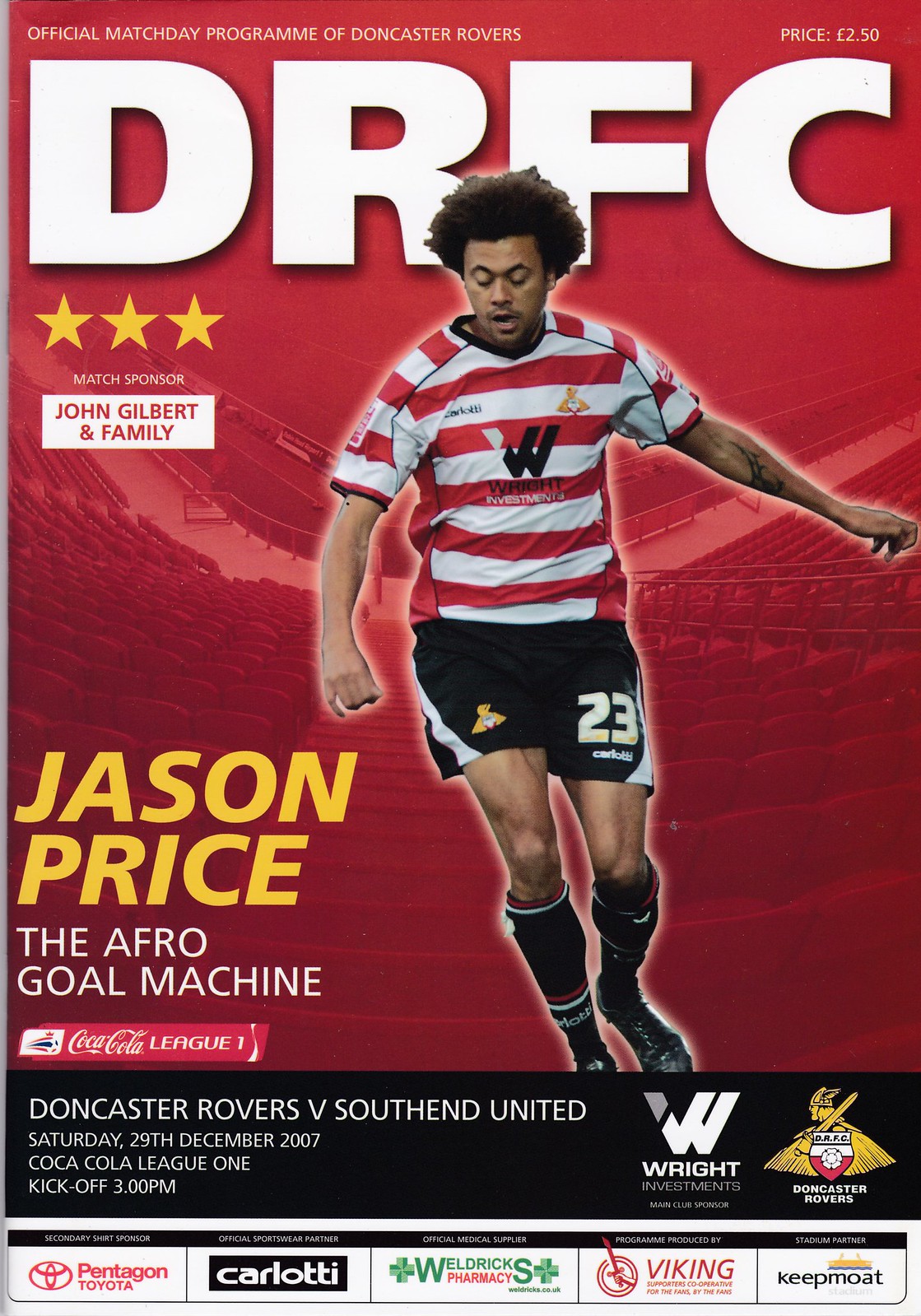The cover of the official match day program for Doncaster Rovers, priced at £2.50, prominently features the title "DRFC" in bold white letters. The cover showcases an image of Jason Price, dubbed "The Afro Goal Machine," a black soccer player donning a red and white horizontally striped shirt, black shorts, knee-high socks, and sports shoes. He is pictured looking down, likely towards the ball. The program also highlights that the match is sponsored by Jim Gilbert and family. Additionally, there's information about the match between Doncaster Rovers and Southend United, scheduled for Saturday, 29th December 2007, with a kickoff time of 3 p.m. This match is part of the Coca-Cola League One. Logos for various sponsors, including Pentagon, Toyota, and Carlotti, are displayed at the bottom of the cover.